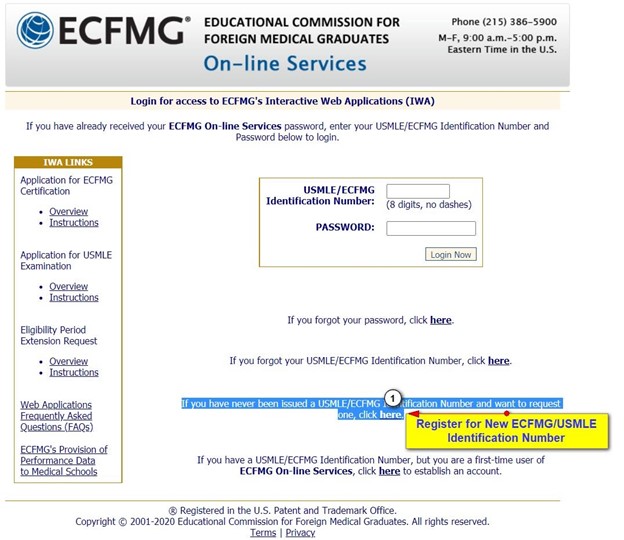The image features a clean white background with a blue header prominently displaying "ECFMG," which stands for the Educational Commission for Foreign Medical Graduates. Beneath the header, in blue text, it reads, "Online Services," followed by a contact phone number: (215) 386-5900. The available hours for phone support are listed as Monday to Friday, 9 a.m. to 5 p.m. Eastern Time in the U.S.

Below this information, instructions are provided to log in to ECFMG's Interactive Web Application (IWA). It advises users who have already obtained their ECFMG online services password to enter their USMLE/ECFMG identification number and password in the fields provided. The identification number field specifies that it should be an eight-digit number without dashes. 

Adjacent to the input fields for the identification number and password, there is a beige rectangular button labeled "Log In Now." Additionally, a link is provided for users who have forgotten their password, with the word "here" emphasized in bold. If you have forgotten your USMLE/ECFMG identification number, further instructions are indicated but not fully detailed in the image snippet.